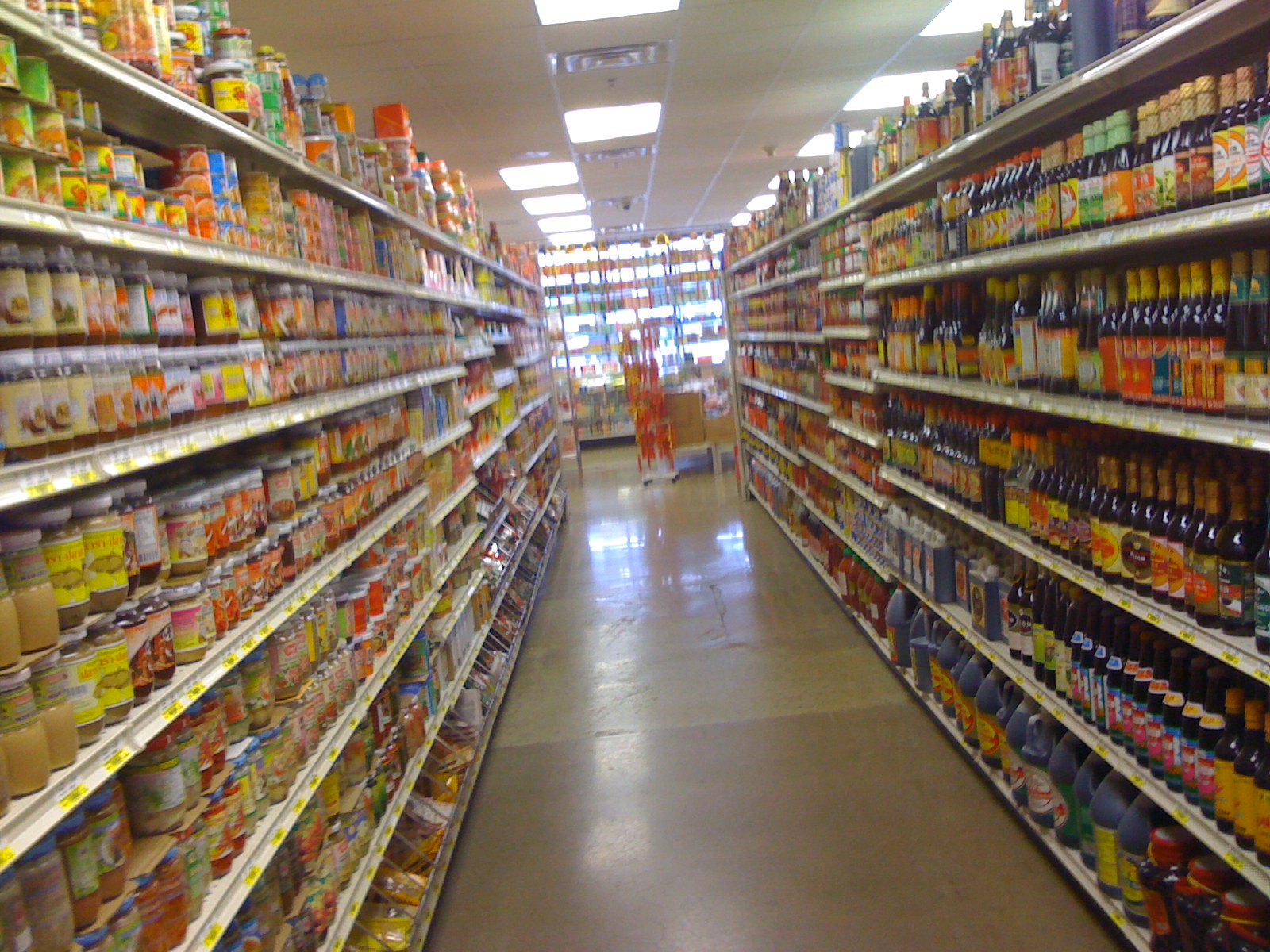A candid, slightly blurry photograph captures the bustling ambiance of a small supermarket aisle, presumably while the photographer was in motion. The setting resides in a section dedicated to world foods, with shelves densely packed on either side. Dominating the right side are numerous small bottles filled with a dark liquid, likely soy sauce, their vibrant labels vividly contrasting against one another. These labels showcase a rich amalgamation of colors—yellows, oranges, reds, and golds—giving the frame a lively, dynamic atmosphere. No text is visible, allowing the myriad of products with their distinct markings to take center stage. Towards the back, a window subtly hints at the world beyond, as the aisle stretches out, revealing the everyday character of this multicultural shopping experience.